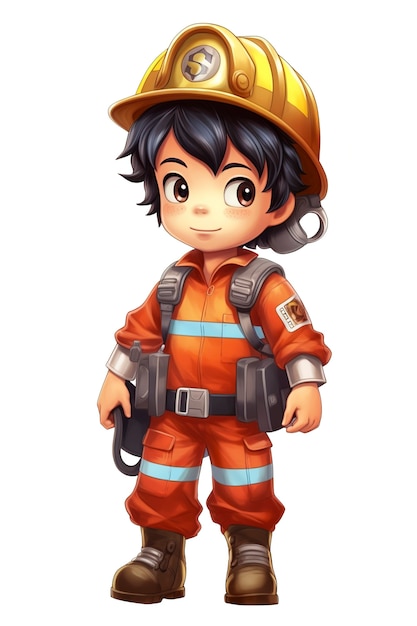This animated image depicts a cute, cartoon firefighter reminiscent of characters from Paw Patrol. The little boy is outfitted in a detailed firefighter's uniform. He wears a yellow and brown hard hat, prominently featuring a circle with an "S" on it, and has black tufted hair with gray highlights. His large brown eyes gaze to the right, set against his white skin. His attire includes an orange fire jumpsuit with a fold-over collar, long sleeves, and a turquoise stripe running horizontally across his chest, as well as around each pant leg. The jumpsuit also features pockets; one on the chest and side flap pockets on the legs. He is accessorized with a black belt and gray suspenders, which appear to be part of a light brown backpack strapped over his shoulders and secured with metallic buckles. Additional details include a white arm patch with orange accents on his sleeve and brown boots completing his ensemble.